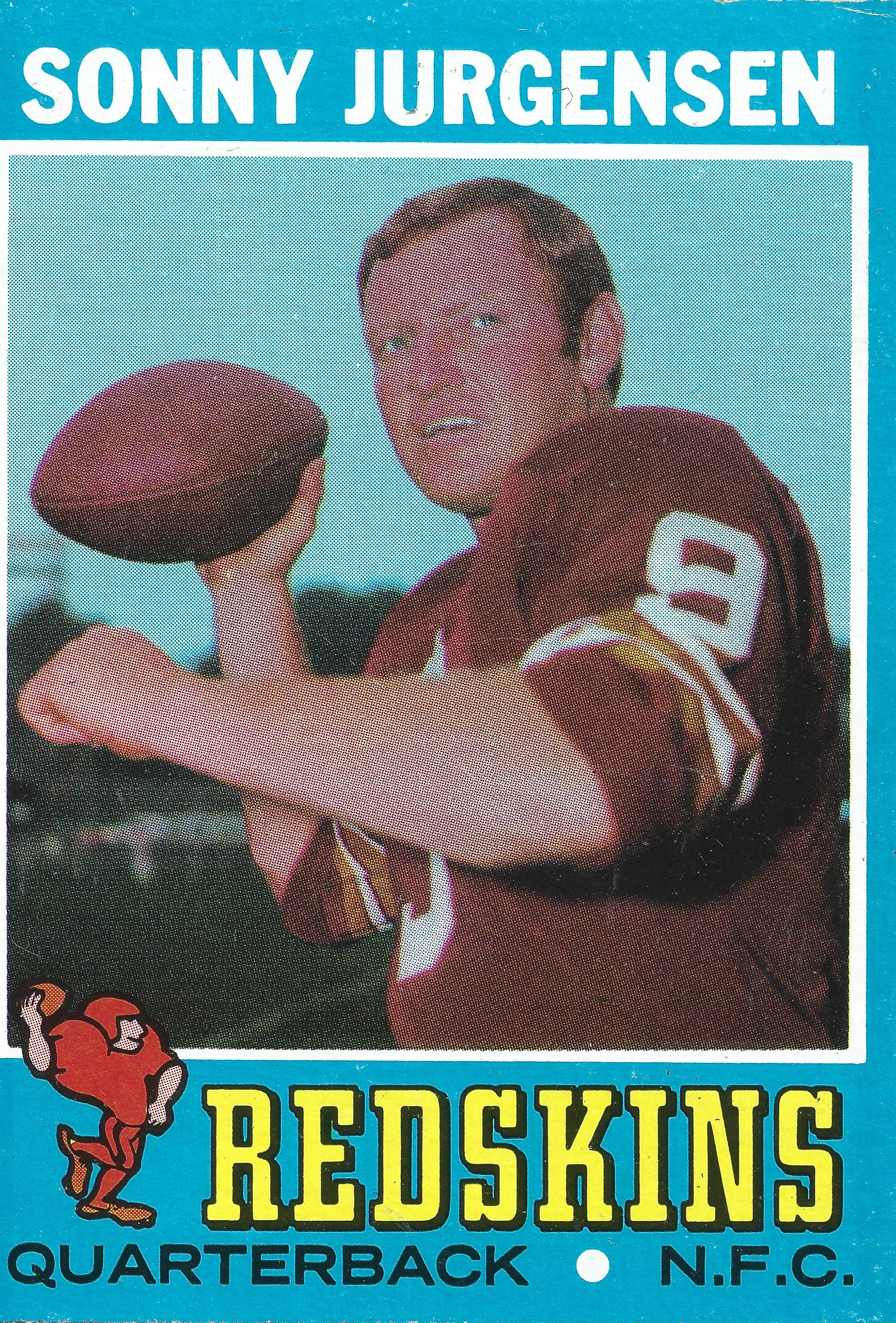The magazine scan features an action photograph of Sonny Jorgensen, poised to throw a football as he gazes off into the distance, targeting his pass. Clad in a brown jersey prominently displaying the number 9 in white, "Redskins" is inscribed beneath the number in yellow lettering, referencing the Washington Redskins team. The background presents a clear blue sky, accentuating the vibrant colors of the image. Above Sonny's head, his name "Sonny Jorgensen" is boldly written in white. Additional elements in the image include a small, exaggerated cartoon illustration of a football player, accompanied by the text "Quarterback NFC" in black, further detailing Jorgensen's position and league affiliation. The composition captures the intensity and focus of a professional game setting.